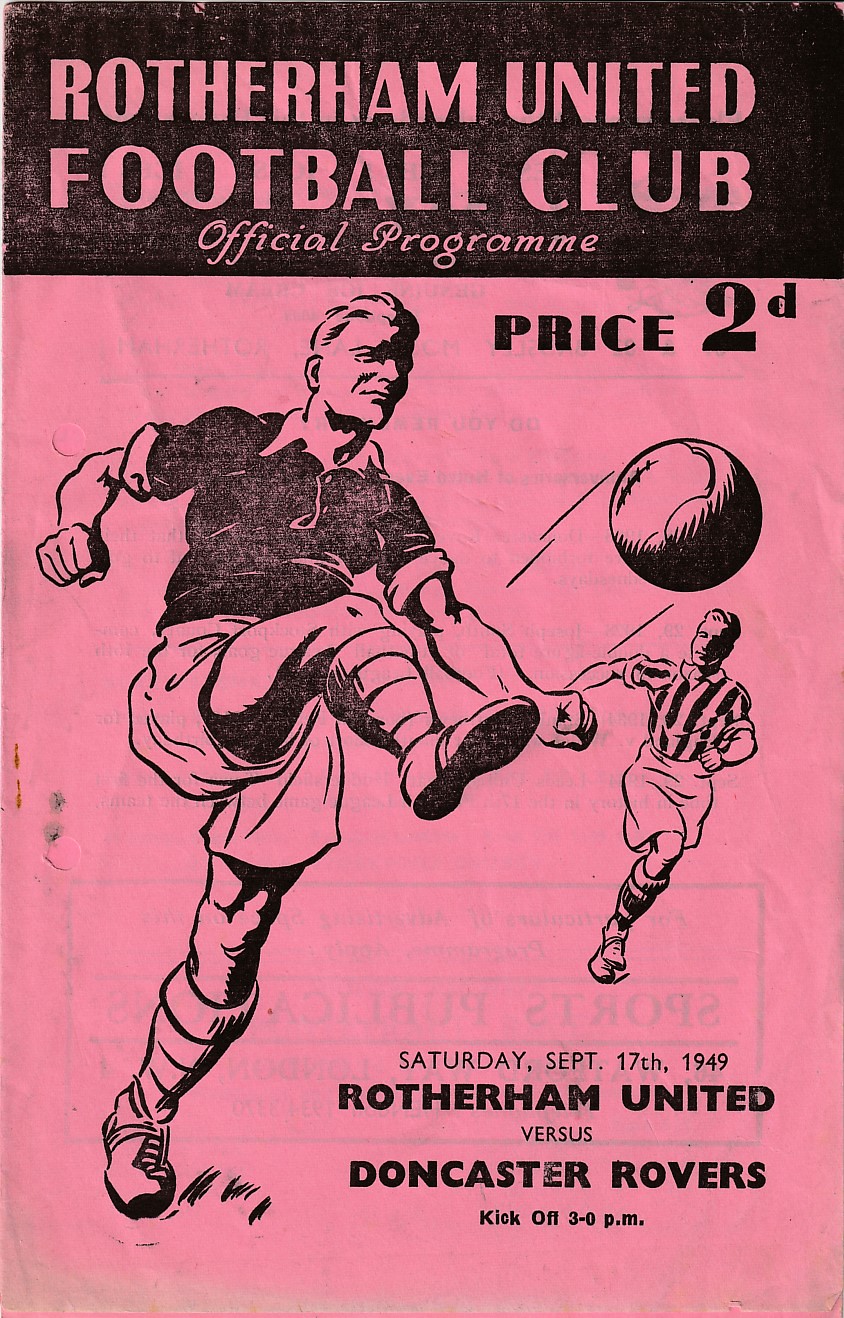This is a vintage poster from the late 1940s, specifically the official program for the Rotherham United Football Club. The horizontally rectangular print piece is bright pink, with a black banner at the top proclaiming "Rotherham United Football Club Official Program, Price 2D." The central illustration features a muscular man, dressed in a dark shirt and white pants with knee-high socks, energetically kicking a soccer ball. A referee, in traditional referee attire, stands nearby. At the bottom, the date "Saturday, September 17, 1949" is prominently displayed, along with details of the match: Rotherham United versus Doncaster Rovers, with kickoff at 3 p.m.